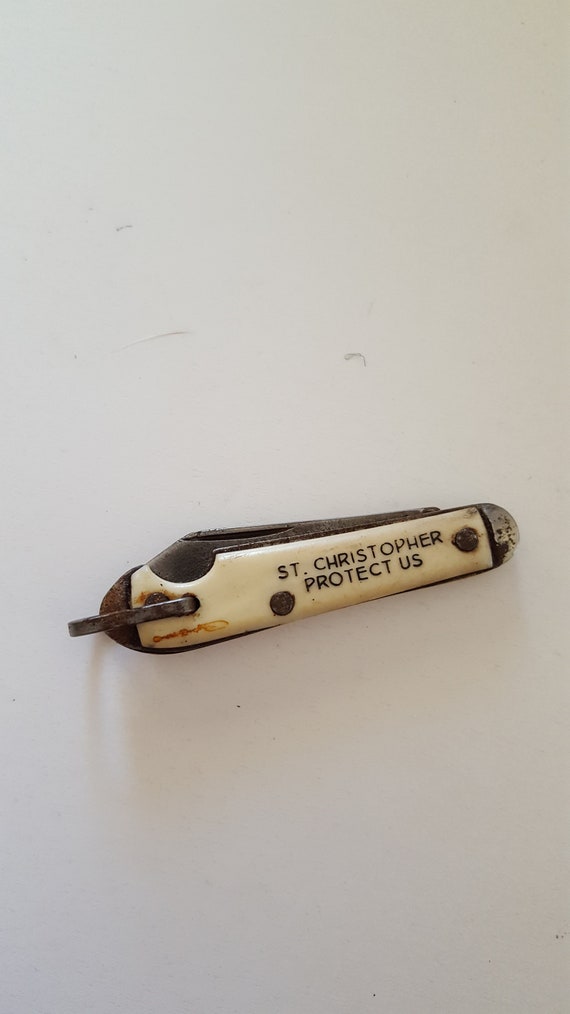This image features a vertical rectangular photograph with a light brownish-white background that fades into gray. In the center rests an old, well-worn pocket knife, placed horizontally at a slight angle, dipping downwards from right to left. The knife has a beige plastic handle that exhibits brown stains and signs of age. Secured with three old-looking and rusted rivets, the handle appears to be attached to a steel mechanism. The top portion of the blade and the tip of the handle both show significant rust.

Engraved on the knife handle are two lines of all-caps black text: "ST. CHRISTOPHER" and below it, "PROTECT US". The inscription is centered and prominent against the stained beige background of the handle. Notably, near the right side, there is a metal half-circle or dome-shaped clip, which is also rusted, indicating that the knife could potentially be attached to a chain or clipped to a belt or pocket. This pocket knife, featuring two blades of different lengths, evokes a sense of historical utility, possibly dating back to an era when Saint Christopher's protection held significance for travelers.